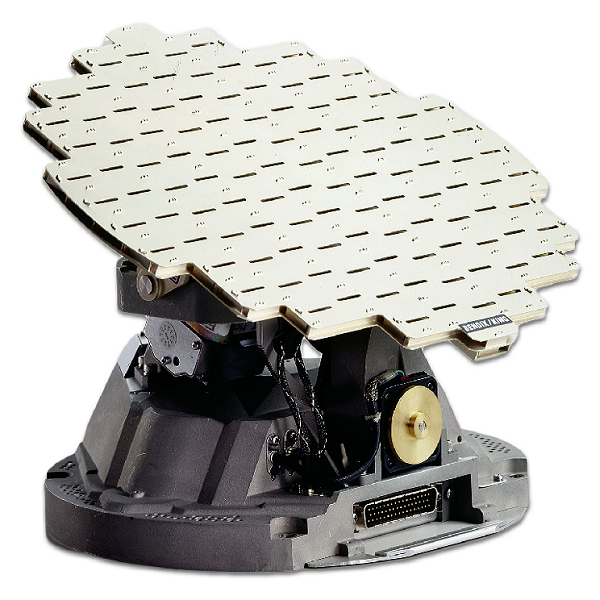The image depicts a small, vintage piece of machinery with a flat, jigsaw puzzle-like metal plate on top, angled downward. The top plate is a lighter, shinier silver metal with etched lines. Below the plate sits a dark gray, gun-metal colored base that features a prominent gear and a gold-colored dial knob. The front of the base has a port with three lines of pins for connecting a plug or cord, indicating electronic components. Additionally, there are visible wires coming from the bottom right-hand side. The overall shape and structure suggest it might be some kind of measurement tool or possibly a component of a larger mechanical system, such as a braking system in a car. The word "king" is partly visible on the machine, though the exact text is unclear. The image is focused purely on the machinery with no background or foreground elements present.